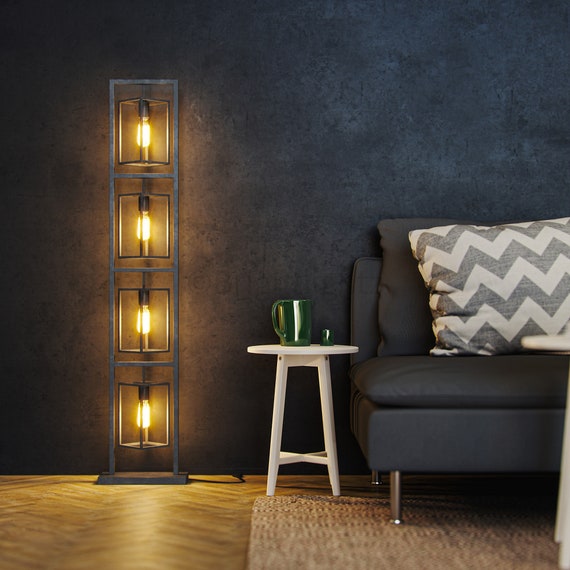A cozy corner of a living room features a sleek, gray armless couch with metallic legs and a pair of decorative throw pillows, one adorned with white and gray zigzag patterns and the other solid gray. The couch rests on a woven, tan and white throw rug that lies atop a parquet wood floor, arranged in an intricate V-shaped pattern of varying tan shades. Adjacent to the couch on the left is a small, round white wooden table topped with a green mug. Anchoring the scene is a distinctive, tall lighting fixture with a gray metal frame, featuring four vertically aligned cylindrical bulbs. The backdrop is a two-tone gray wall, adding depth and contrast to the setting.